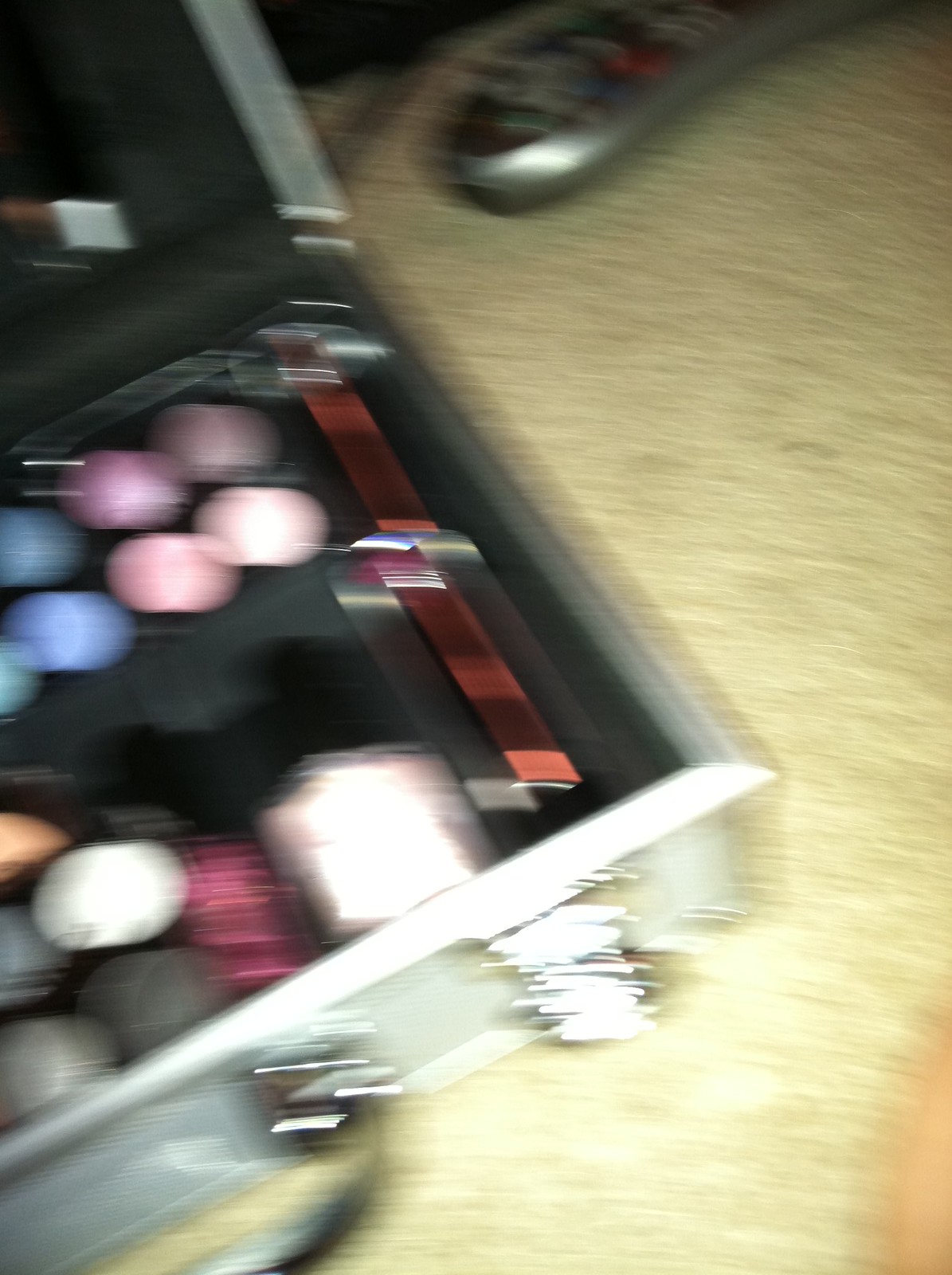This is a very blurry image showing the right edge of a silver briefcase resting on a tan carpet. The briefcase appears to be open, revealing an assortment of colorful items inside, possibly makeup palettes or paint. Specific colors visible at the top of the case include light purple, light pink, darker purple, darker pink, shimmery blue, and blue in circular forms. Additionally, the interior right corner of the case holds two red rectangular objects. On the bottom, although indistinct, there are a white and black circle, along with a dark gray and lighter gray circle in the bottom left of the photo. The upper center of the photo features the edge of a remote control, and the bottom right corner contains either a finger or a knee. The overall composition is blurred, likely due to the motion at the time the photo was taken, making it challenging to definitively identify all the objects.